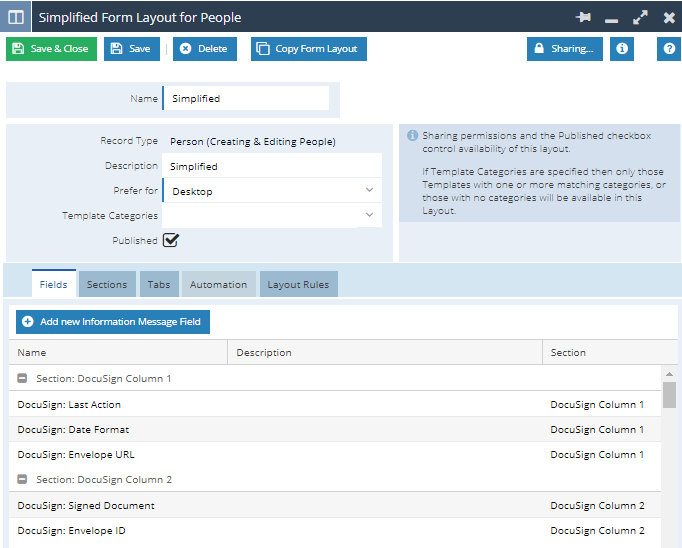The image is a screenshot of a user interface designed for managing form layouts. At the very top is a dark blue header that reads "Simplified Form Layout for People" in light blue text. In the upper right corner of the header, there are two icons: a white 'X' for closing the interface and a pushpin for pinning it.

Below the header, on a white background, there is a row of buttons stretching from left to right. The first button is green and says "Save and Close" in white text. Next to it is a blue button labeled "Save." Following the "Save" button, there is another blue button marked "Delete." Then there's a button labeled "Copy Form Layout." Completing the row are a "Sharing" button and an "Information" button.

Further down, there is a light blue form. Within this form, several fields are present: 

1. A request for the user's name.
2. A description field.
3. A dropdown menu labeled "Prefer For."
4. Another dropdown menu labeled "Template Categories."

Below these fields, the word "Publish" is displayed with a checkbox to its right. To the right of the "Publish" option, there is a note in gray text that says, "Sharing permissions and the publish checkbox control availability of this layout."

This detailed, step-by-step description captures the entire layout and various functional components present in the screenshot.